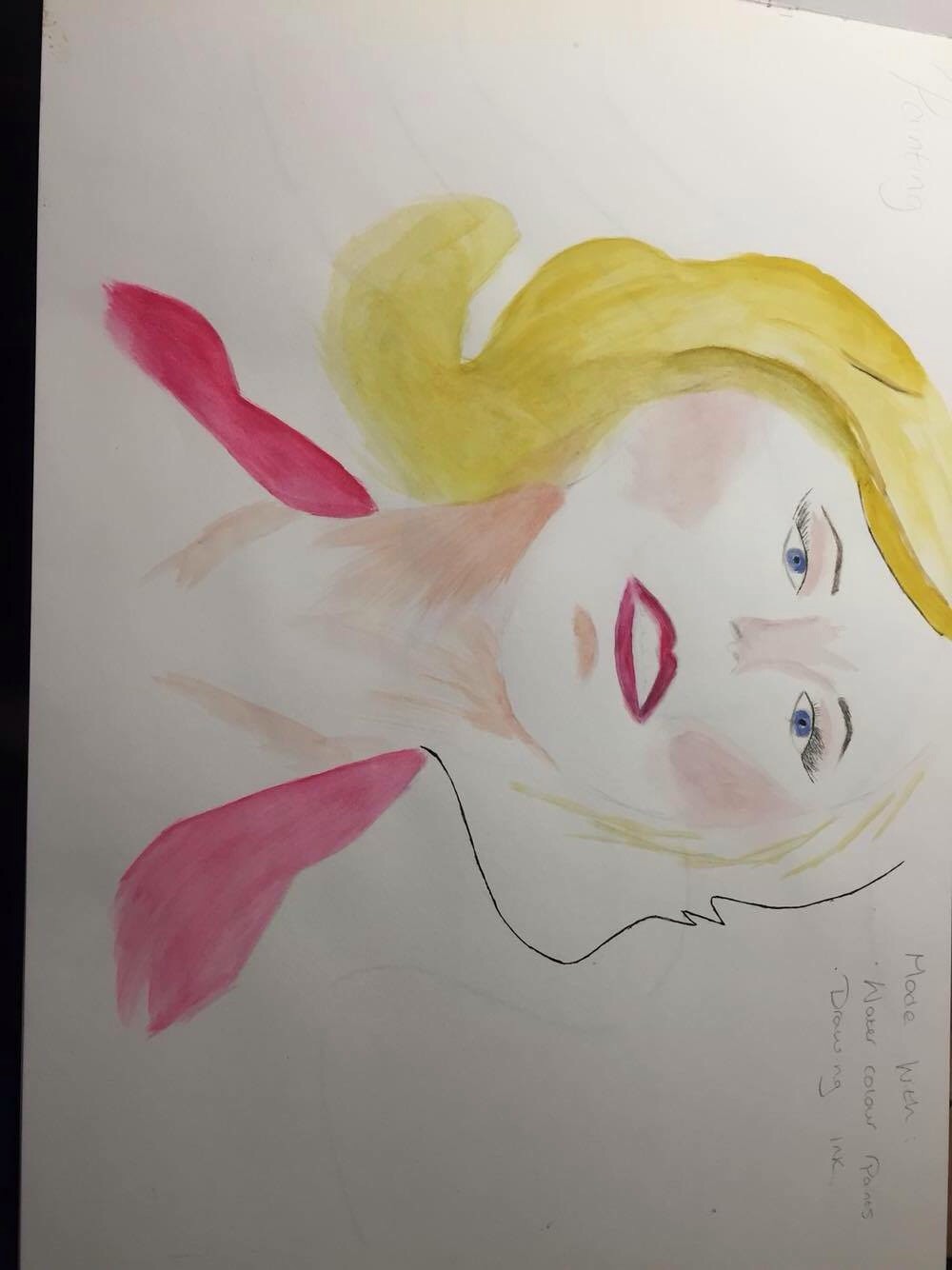This is a detailed watercolor portrait of a blonde woman, depicted on a white sheet of paper tilted 90 degrees from its intended orientation. The woman appears to be in her 20s or 30s with a haughty expression, characterized by a look of disdain and disgust. She has striking blue eyes and wears bright red lipstick on her open mouth. Her long blonde hair sweeps over the right side of her head, while the left side seems less detailed. She is adorned in a red cape or possibly a scarf that outlines a low-cut or V-cut blouse. The artwork includes extensive writing, although it's mostly illegible. In the upper right corner, it faintly reads "mode with watercolor paints, drawing ink." The portrait emphasizes her slender neck and thin nose, further enhancing her aloof demeanor.